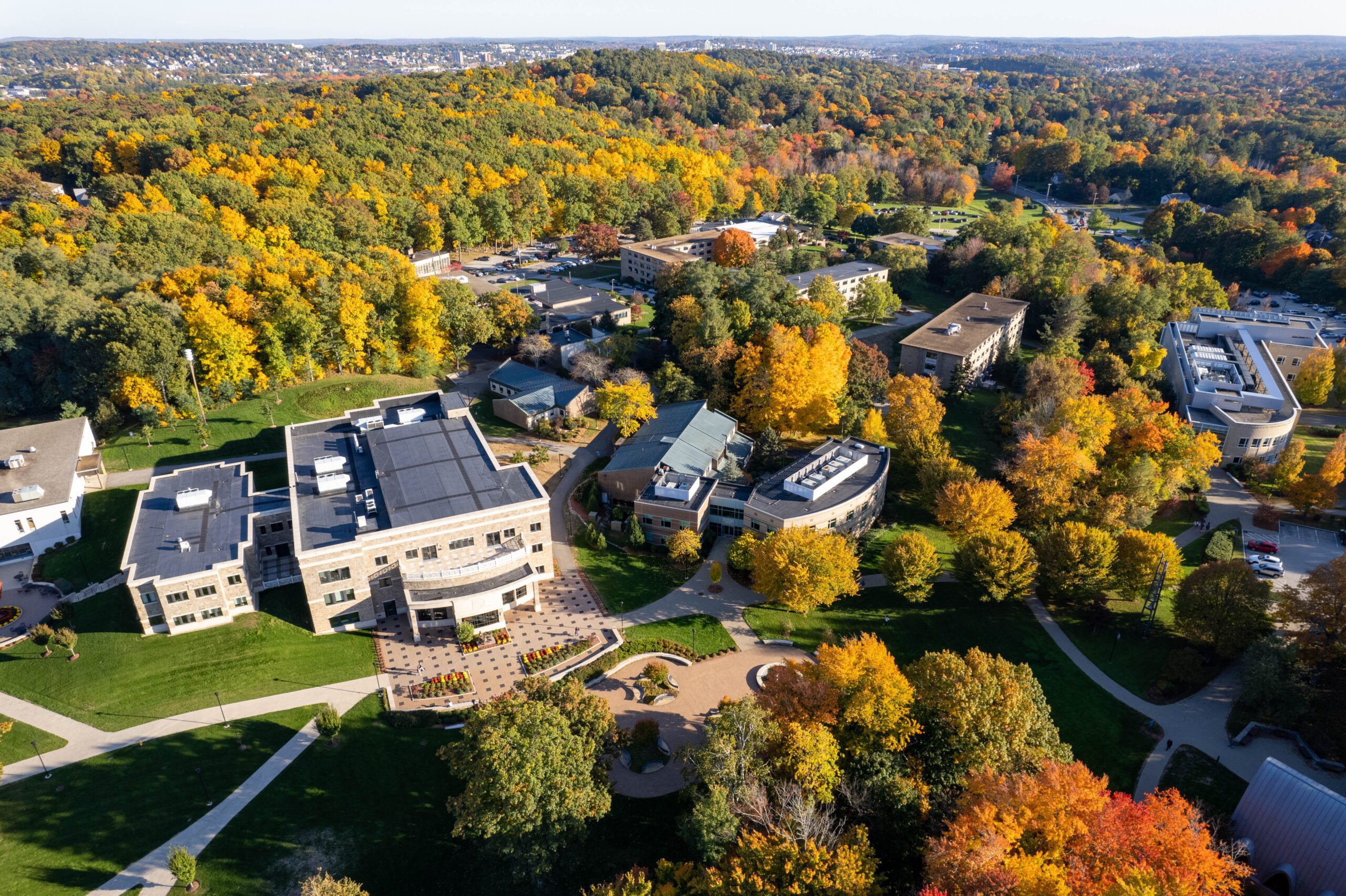The photograph presents a contemporary aerial view of a residential complex nestled in a hilly, forested area with deciduous trees in various stages of autumn color. In the background, beyond the forested hills, the faint outline of a cityscape suggests a distant urban area. The residential complex, potentially comprising upper-scale apartment buildings, condos, or vacation villas, is centrally positioned. The buildings are primarily white with flat roofs, adorned with patios and connected by an intricate network of concrete walkways. Some of the roofs house white air conditioning units. The largest building, situated in the center-left and standing three stories tall, features a prominent patio and is connected via a walkway to an adjacent two-story structure, highlighting the complex's spread-out design. The foreground features a mix of red, yellow, and green tree tops, enhancing the autumnal scenery. The overall setting, with ample greenery and minimal visible parking, suggests a tranquil, well-planned residential area embraced by nature.